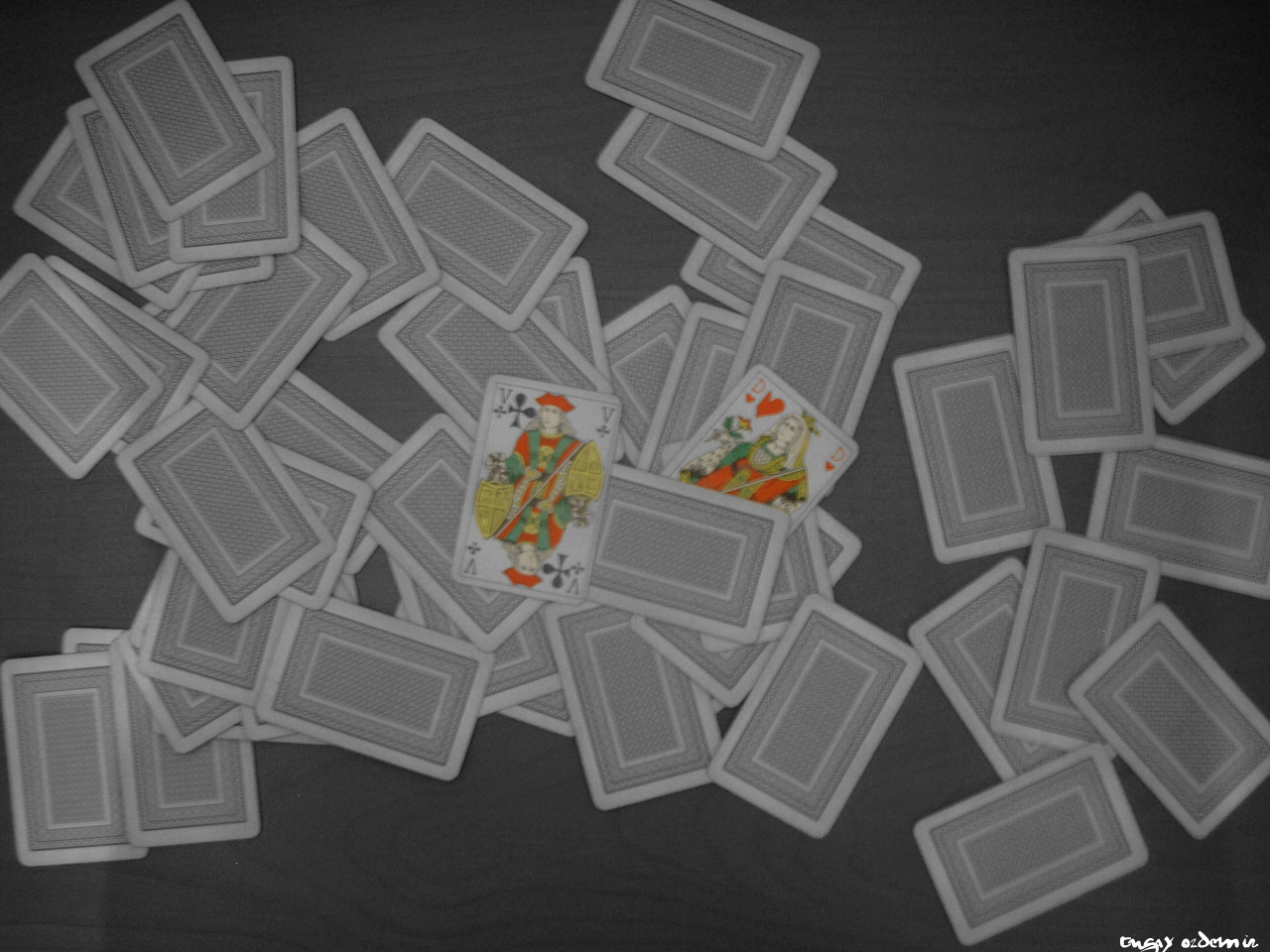This image, captured by photographer Onse Ozdemia, is a striking example of product photography with a focus on playing cards. Staged against a deep black background, the composition features a chaotic yet artistic arrangement of playing cards scattered across a similarly dark-colored carpet. The cards are positioned at various angles and layered over one another, creating a sense of dynamic disarray.

Among the jumbled cards, two are particularly noticeable. One card prominently displays the letter "V" and features the illustration of a Queen of Hearts, while another showcases the letter "D" along with an image of a King of Clubs. The "V" card is fully visible, whereas the "D" card is partially obscured by another card.

The photographer’s signature, "Onse Ozdemia," appears in white at the bottom right corner of the image, adding an elegant finishing touch to this dramatic and meticulously detailed product shot.